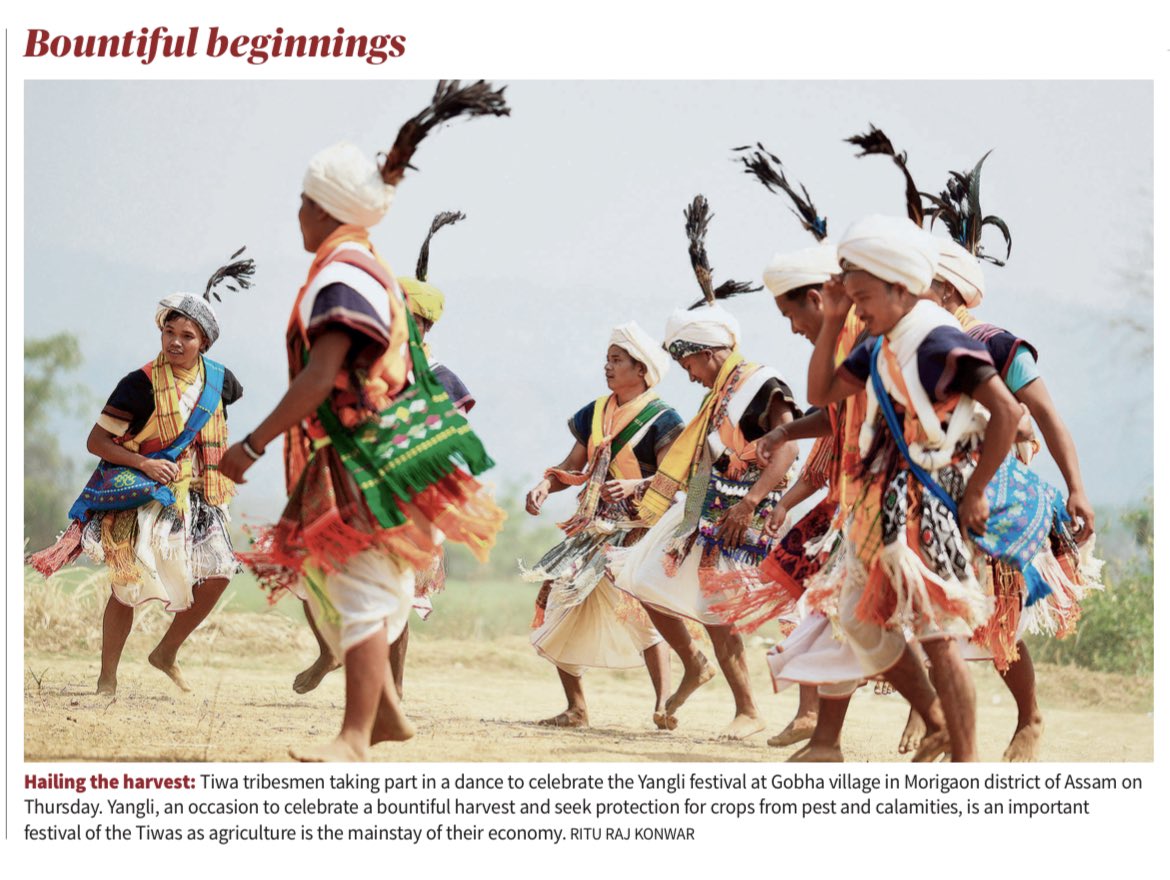The image appears to be a poster or magazine page set against a blue sky background with earthy soil and foliage. The title "Bountiful Beginnings" is prominently displayed at the top in an italic red font. The scene below features several Tiwa tribesmen energetically participating in a traditional dance celebrating the Yangli festival at Copa village in Morigaon district of Assam. These men are dressed in elaborate, multicolored vests, white turban-like hats adorned with long black feathers, and skirts. Each dancer, barefoot with tan skin, carries a differently colored bag over one shoulder. They are all captured mid-dance, with their feet in the air, highlighting the vibrancy of their movements. The bottom of the image reads "Hailing the Harvest" in red, followed by a caption explaining that the Yangli festival is a significant agricultural celebration to ensure a bountiful harvest and protect crops from pests and calamities. The caption includes attribution to Ritu Raj Kanwar.